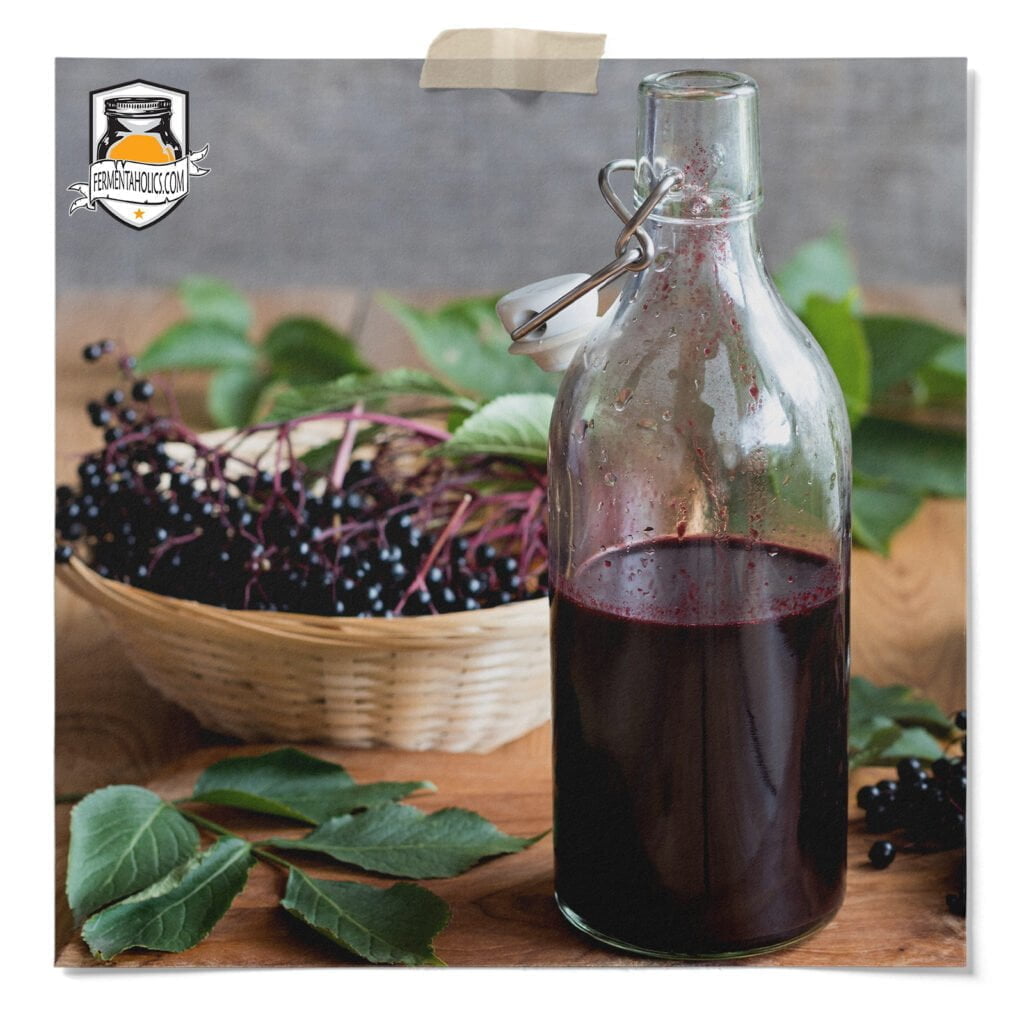In this perfectly square image, a light tan wicker bowl filled with grapes is prominently featured. The deep purple, almost black grapes, still attached to their red vines, share the bowl with scattered green leaves, all resting on a wooden table. In the foreground to the right, a clear glass filled halfway with very deep red wine adds a rich contrast. Additional leaves and grapes are artfully strewn across the table surface. The background is a solid gray, providing a neutral backdrop that highlights the vivid colors in the foreground. In the upper left corner, a mason jar logo with an orange semicircle and white shield mark the brand Fermentaholics.com. Over the top edge of the picture, a piece of brown tape is visible, adding a rustic touch to the composition.